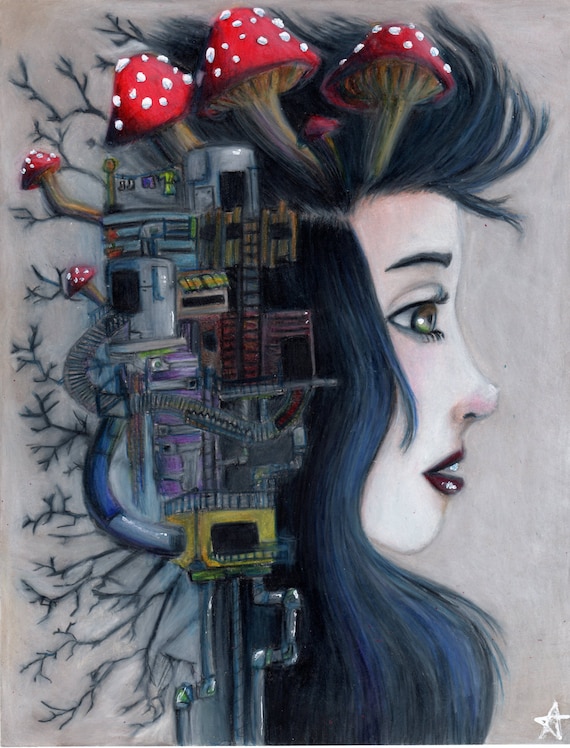This vertical artistic image features a side profile of a pale-skinned woman with striking green eyes, long black hair accented with blue, and maroon-colored, glossy lips, slightly parted as she gazes into the distance. Her hair, drawn with intricate details, flows down her right side and exhibits both organic and mechanical elements. From her windswept bangs sprout red and white speckled mushrooms, whose stems blend into her hair. Below these mushrooms, a complex structure, resembling a dystopian fire escape or tower, intertwines with her hair. This structure, complete with stairs, slides, and tin can-like homes adorned with hanging clothes, gives off a science fiction vibe. Additionally, tree-like black roots and mechanical gears, pipes, and gold-accented boxes emerge from her hair. Set against a grayish background, the artist's signature white star is displayed prominently in the bottom right corner.